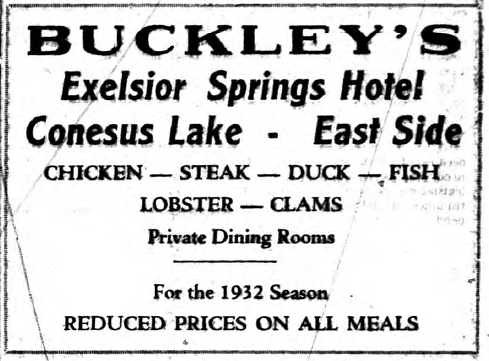This image is a vintage black-and-white advertisement, resembling an old flyer or newspaper clipping, printed on creased white cardstock with a black, ink-smeared border. At the top, "Buckley's" is prominently displayed in large black letters, followed by "Excelsior Springs Hotel" and "Conessus Lake, East Side". The middle section lists menu items in a smaller font: "Chicken, Steak, Duck, Fish, Lobster, Clams." Below this, "Private Dining Rooms" is noted, and at the bottom, it announces, "For the 1932 season, reduced prices on all meals." The overall condition of the card suggests it's nearly a century old.